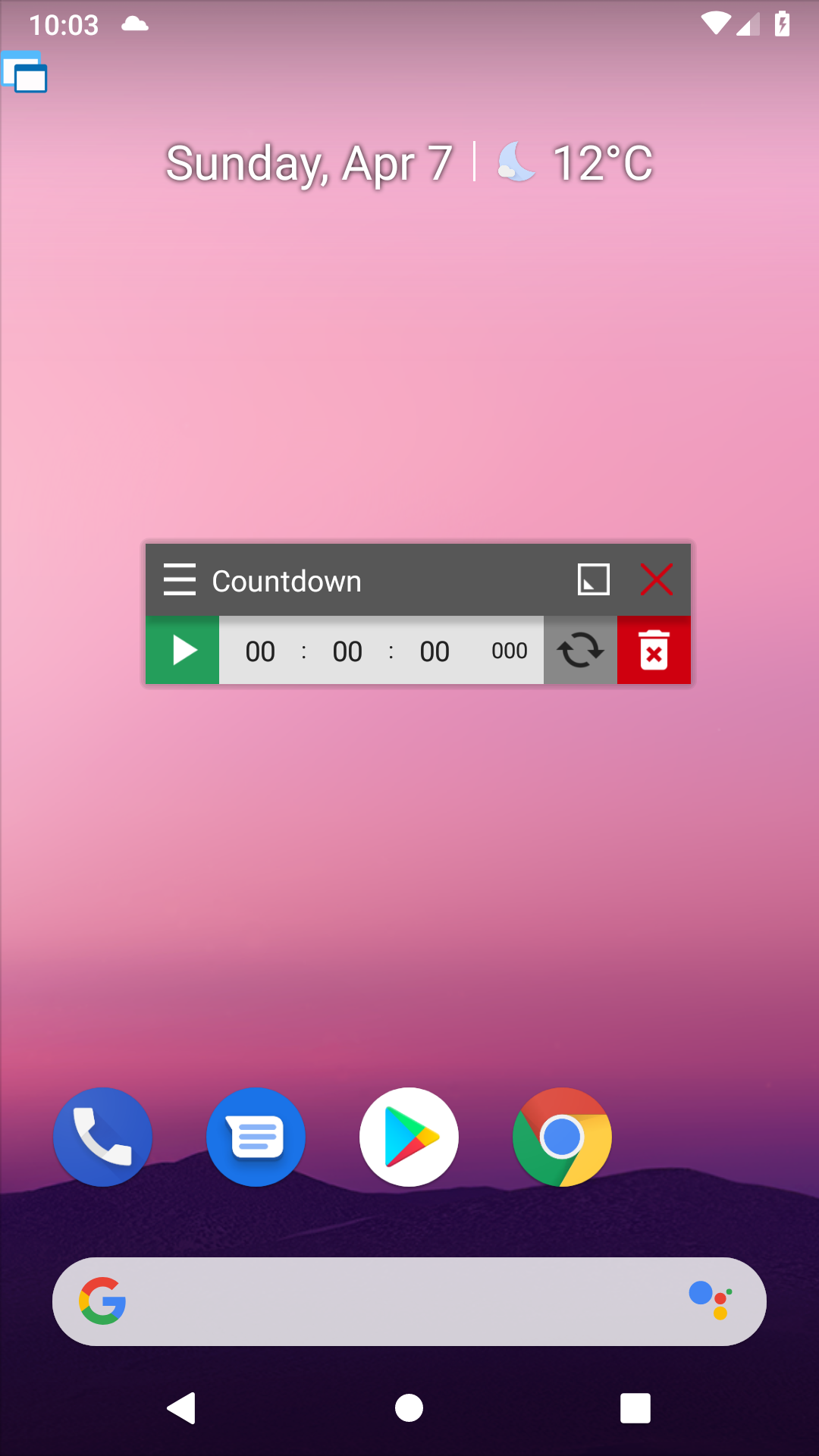The image is a vertical rectangular area with a gradient background transitioning from light pink at the top to light purple, then dark purple, and finally black at the bottom. 

In the top-left corner, the time is displayed in white as "10:03," and to the right is a white battery icon. Below the time on the left side are two small, white rectangular images resembling computer screens; the one behind has a turquoise top, and the one in front has a dark top.

Centered on the page in white font are the words "Sunday, APR 7," followed by a vertical line, a moon with a small cloud, and "12°C" indicating the temperature. 

Midway down the page is a horizontal rectangular section with a gray top bar. On the left are three horizontal lines, the word "countdown" in white, and a red 'X' on the far right. Below this section is a vertical green rectangle with a white triangle pointing right, displaying "00:00:00" and three zeros, flanked by two arrows indicating a circular motion. Adjacent to this green area is a red section with a white trash can icon and a red 'X.'

In the lower quarter of the screen, there are four circles: a blue one with a white telephone icon, a turquoise one with a white paper and three horizontal lines, and two multi-colored circles. 

Below these circles is an oval, horizontal box with a colorful Google "G" on the left and colored elements on the right. Finally, in the dark section at the bottom, there are three white icons: a triangle pointing left, a circle dot in the center, and a square on the right.